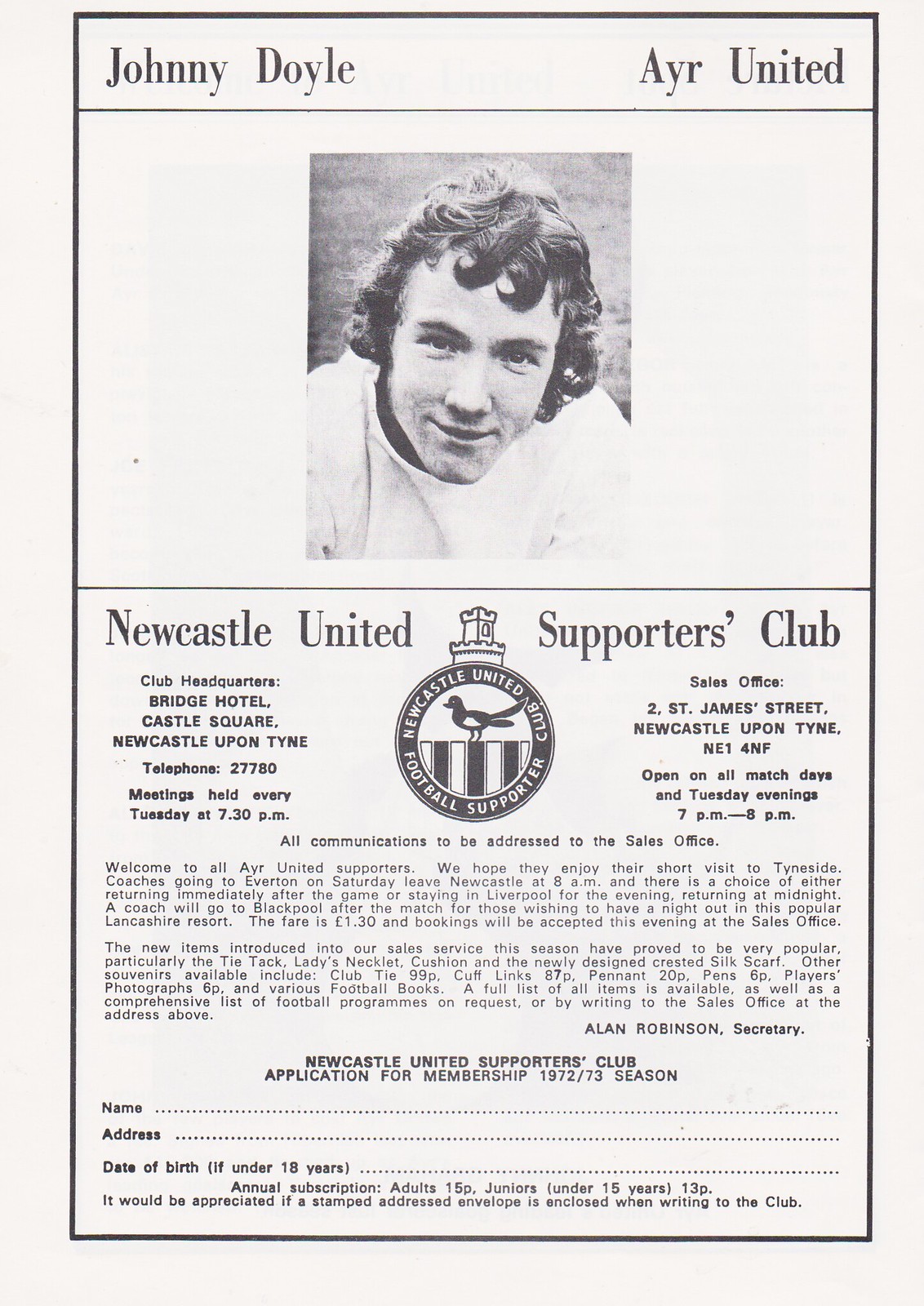This black and white image appears to be a page from an old British football magazine, serving as both an advertisement and a membership application for the Newcastle United Supporters Club for the 1972-73 season. At the top left corner, in bold black text, it says "Johnny Doyle," while the top right corner reads "AYR United." Below this, centered on the page, is a headshot of a smiling white man, presumably Johnny Doyle. Directly beneath the photo, in prominent black letters, is the title "Newcastle United Supporters Club." 

The page is bordered in black and features a circular club logo in the middle, depicting white and black bars, with a black bird and a castle turret, accompanied by the text "Newcastle United Club Football Supporter." To the left of the logo, the club headquarters' address, telephone number, and operating hours are displayed. On the right side are the sales office details, including an address, telephone numbers, and operating hours. 

In smaller text below these sections, it notes communications should be addressed to the sales office, on behalf of Alan Robinson's secretary. Towards the bottom of the page, the text "Newcastle United Supporters Club, application for membership" is followed by lines for "name," "address," and "date of birth," inviting fans to apply for the club's membership.